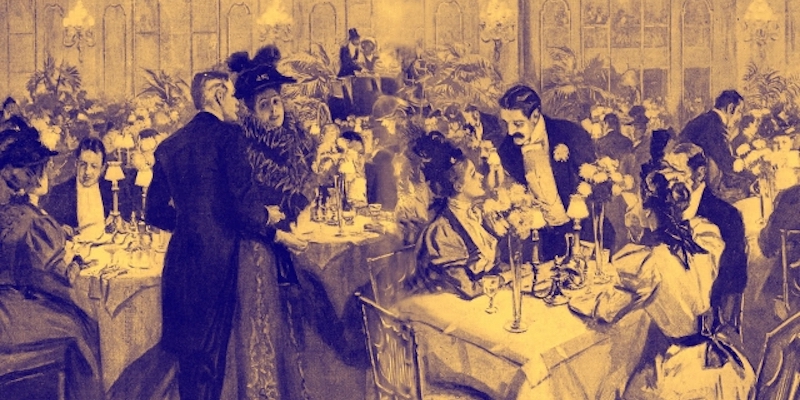This sepia-toned, hand-drawn piece of art captures a high-class gathering in a large, ornate room from the early 1900s. The scene is filled with elegantly dressed men in tuxedos and suits and women in flowing, elaborate dresses and formal headdresses. Numerous tables, set with vases of white flowers, wine glasses, and dishes, are scattered throughout the room. Guests are seen milling about, enjoying dinner and drinks, and engaging in lively conversation. Waiters in tuxedos move gracefully, attending to the patrons. In the forefront, a couple stands out—a woman in a fur coat with a fancy hat and a man seen from behind, also in formal attire. The background reveals intricate details such as chandeliers and ornate wall lighting. Adding to the period charm, there are potted plants and hints of large trees subtly integrated into the scene, alongside people standing or seated, all contributing to the lively, sophisticated atmosphere of the event.